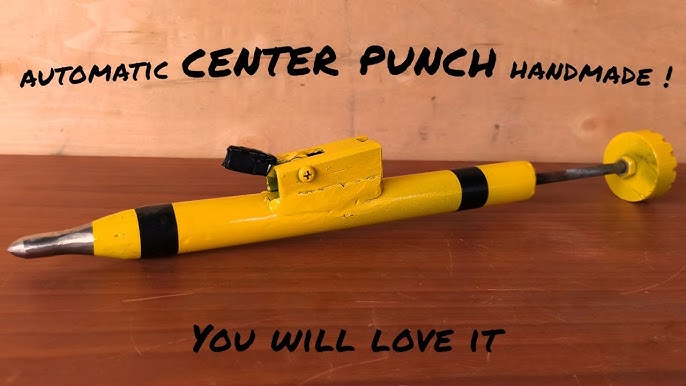The image depicts a handmade Automatic Center Punch displayed on a dark brown wooden table against a light brown, pink-orange particle board background. At the top of the picture, in bold black, handwritten-style text, it reads "Automatic Center Punch Handmade!" and at the bottom, in similar black text, "You Will Love It."

The center punch itself is prominently featured in the middle of the image. It is primarily yellow with alternating black and yellow stripes. On the left side, it has a sharp silver point, while the body of the punch comprises a tubular yellow cylinder. Attached to the cylindrical body is a small trigger mechanism, secured with a screw and resembling a mini handle or bracket. The back end of the punch has a push plunger, also in yellow, which can be activated to force the punch. This detailed design suggests careful craftsmanship and robust construction, emphasizing its handmade quality.